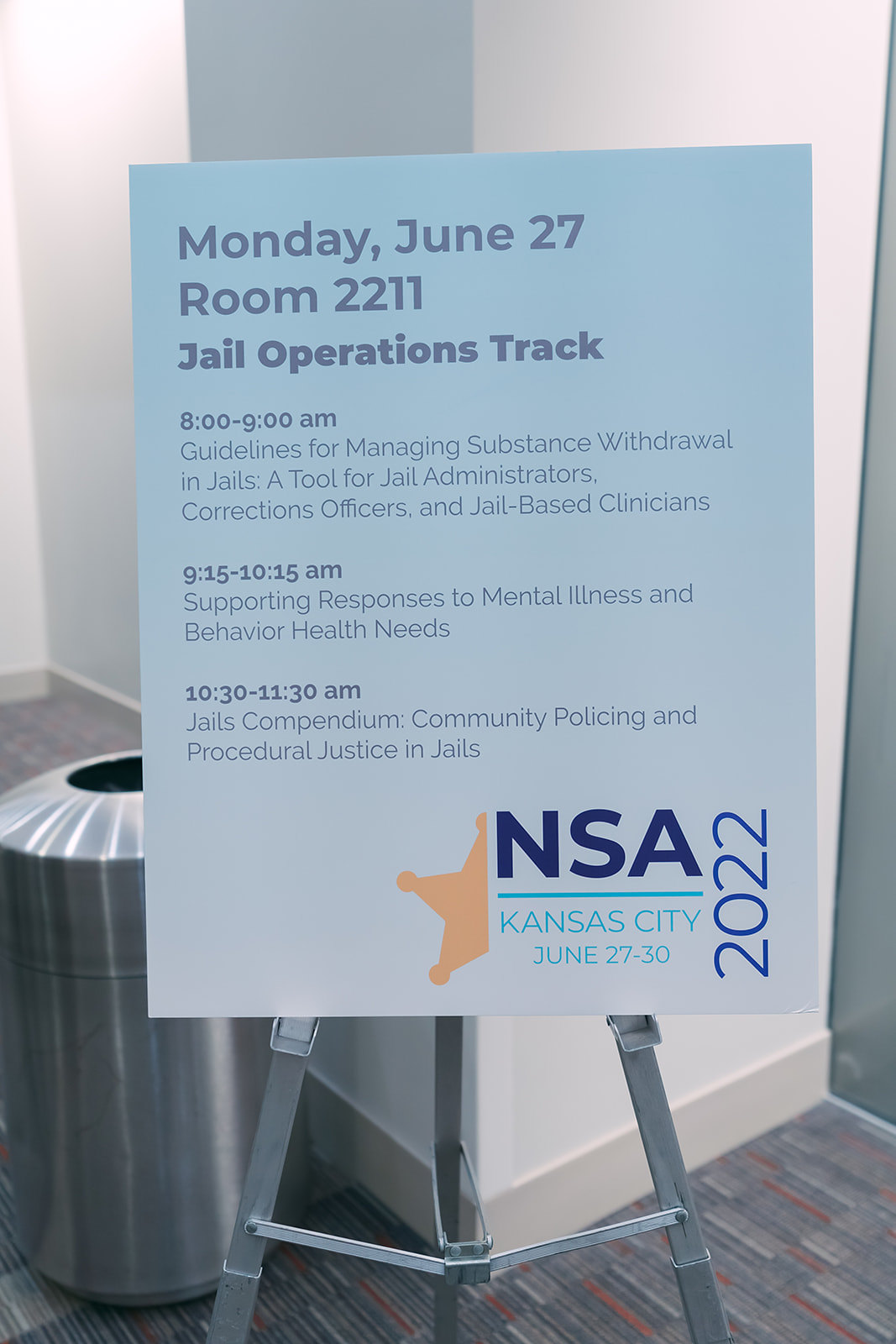The image depicts a light blue to off-white gradient sign on a silver tripod easel, standing on a gray carpet with a striped pattern. The background features a tall white column and a shiny aluminum trash can to the left. The text on the sign is in medium gray and dark blue, displaying detailed information for an event. It reads:

"Monday, June 27th, Room 2211, Jail Operations Track." 

Following this are three sessions:
- "8:00 to 9:00 AM: Guidelines for Managing Substance Withdrawal in Jails — A tool for jail administrators, corrections officers, and jail-based clinicians"
- "9:15 to 10:15 AM: Supporting Responses to Mental Illness and Behavioral Health Needs"
- "10:30 to 11:00 AM: Jails Compendium — Community Policing and Procedural Justice in Jails."

In the lower right corner of the sign is a logo featuring the left half of a sheriff’s badge in dark yellow, with "NSA" written next to it. Beneath "NSA", vertically oriented text states "2022", followed by "Kansas City", and "June 27th to 30th."